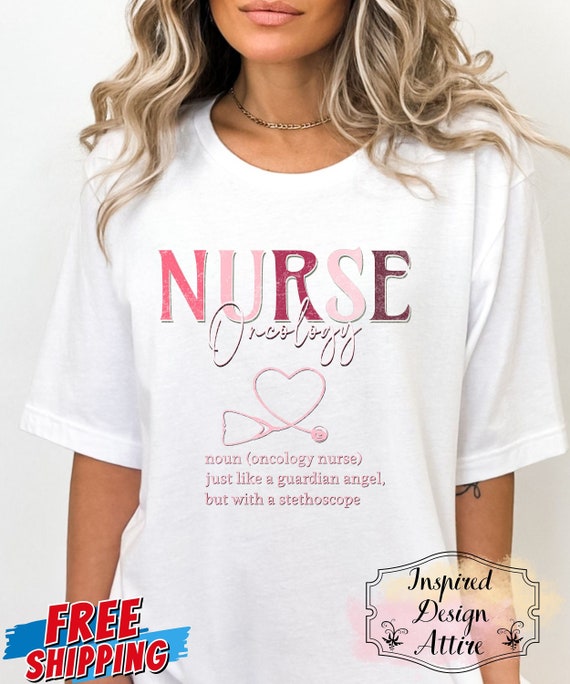This detailed indoor color photograph serves as an advertisement for a t-shirt from Inspired Design Attire. The primary focus is a young woman, approximately 20 years old, visible only from her lips down. She has long, slightly curly hair with alternating shades of blonde and brown, cascading below her shoulders. She sports a short gold chain necklace. The woman is wearing a loose-fitting white t-shirt with the following detailed design prominently displayed on it:

In the center, the word "NURSE" is printed in all capital letters, using various shades of pink—ranging from light to medium and darker pink. Below that, the word "ONCOLOGY" appears in cursive white letters. The design also includes a pink stethoscope with its cord creatively shaped into a heart. Beneath this visual, an inscription reads, "Noun: Oncology Nurse, just like a guardian angel but with a stethoscope," also in different shades of pink.

The bottom left corner of the image features the text "FREE SHIPPING" in bold red uppercase letters, with a blue stripe behind it for contrast. On the bottom right corner, there is the intricate logo of "Inspired Design Attire," displayed in ornate black line art.

The background of the photograph is kept plain and white, ensuring that the t-shirt and its detailed design remain the focal points of this advertising image.